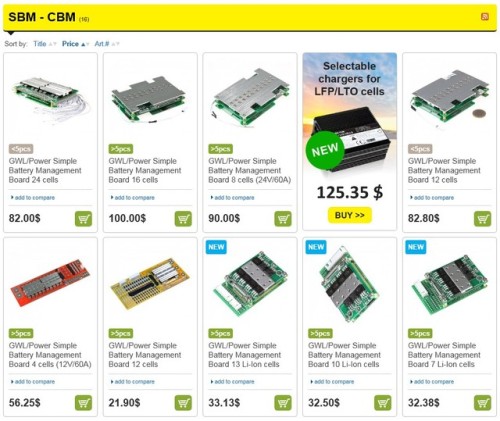The image depicts a webpage showcasing various battery management boards available for purchase. At the top of the page, a yellow banner spans horizontally, displaying the text "SBM-CBM" in bold black letters. Below the banner, it is noted that there are 16 results available. On the right side of the banner, there is a red icon featuring stylized waves emanating from it.

The search results are listed underneath, with sorting options available at the top. The sorting criteria include "Title," "Price" (highlighted with an up arrow), and "Art Number," though the latter is somewhat difficult to discern. The search results are arranged in two rows, each row containing five items.

Each item in the rows features an image of a battery management board, specifying the number of cells it supports, accompanied by its price. Notably, the price format lists the numerical value followed by a dollar sign (e.g., "82.00$"). To the right of each item, there is a green "Add to Cart" button. In the first row, there is an additional section where selectable chargers for LFP and LTO cells or models "125" and "35" are displayed. 

This detailed layout allows users to efficiently compare and select the appropriate battery management board and related accessories for their needs.